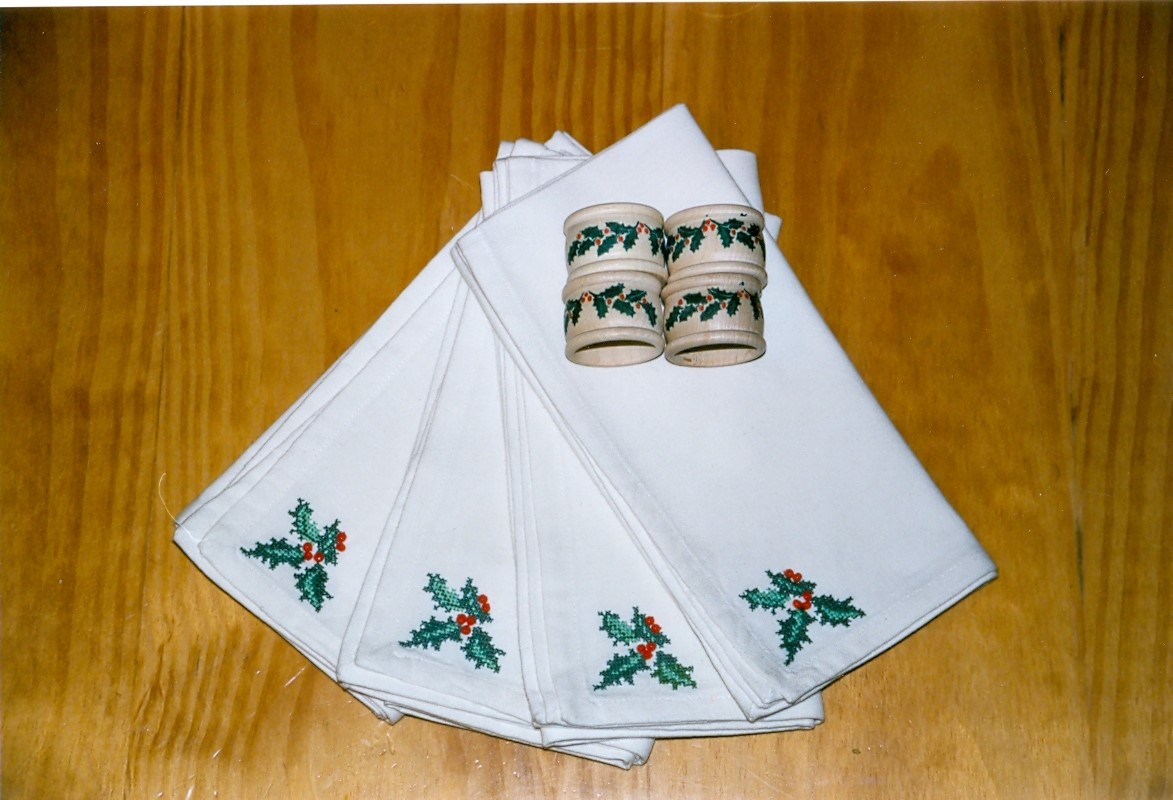This rectangular photograph showcases a festive arrangement of four white napkins, each embroidered with green holly leaves and red berries in the bottom left corner. The napkins are fanned out on a light honey-colored wooden tabletop, emphasizing the rich wood grain texture. Placed atop the napkins are four wooden napkin rings, each adorned with matching holly leaf and berry motifs. The simple yet elegant display highlights both the intricate holiday-themed embroidery and the natural beauty of the wooden elements, creating a warm and inviting holiday setting.